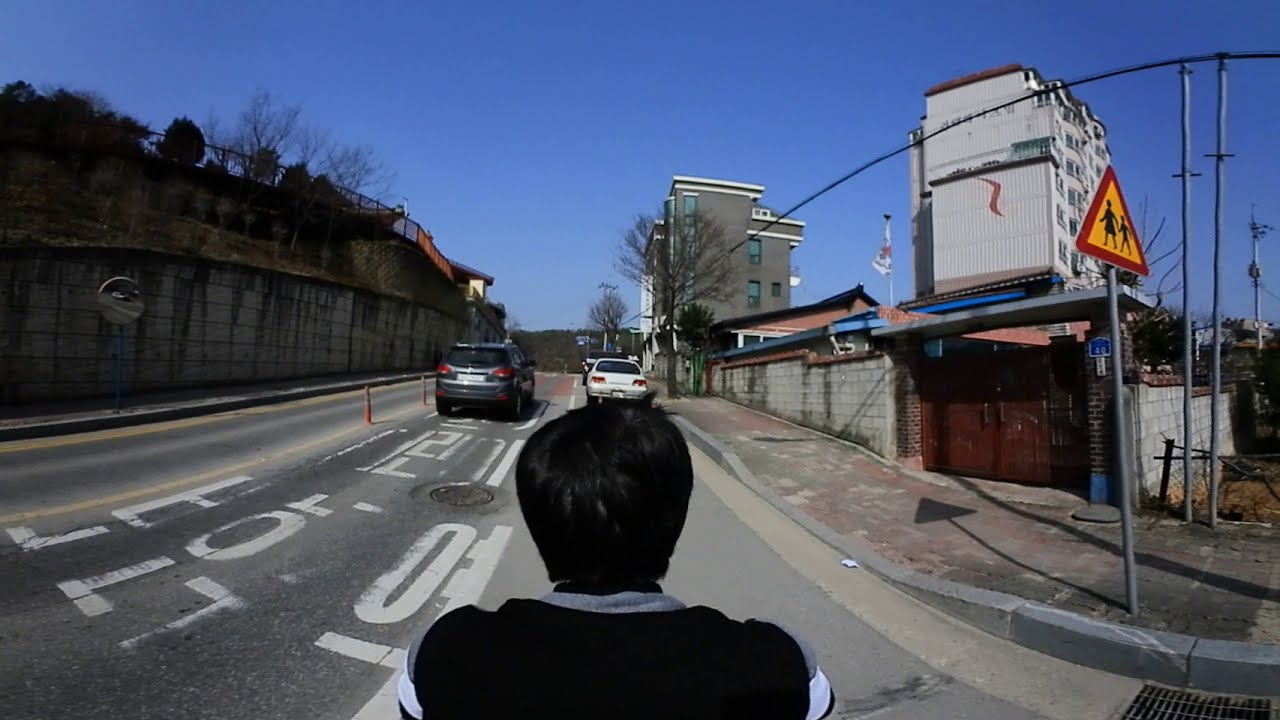In this detailed outdoor photograph, a person with black hair and dressed in a black shirt with gray and white trim is seen from behind, standing or sitting at a crosswalk on a road. The sky above is a clear, vibrant blue with no clouds in sight. To the person's immediate right stands a prominent yellow street crossing sign. 

On the road ahead, there are two vehicles: a gray SUV in motion and a white car parked. To the left of the road, a high retaining wall stretches along, adorned with a mirror. The right side features a small sidewalk accompanied by buildings, among which is a notable Korean flag hinting at the potential location being Korea.

The person appears to be positioned on or near a motorbike, suggesting the photograph might be taken from the perspective of a passenger. The setting is a vivid streetscape combining urban elements with clear navigation markers.